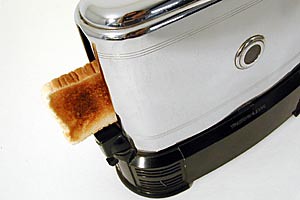This small photograph captures a close-up of a uniquely designed toaster with a piece of toast emerging. The toaster features a distinctive combination of materials and colors: a white body adorned with silver accents and a chrome top, complemented by a black plastic bottom section. A prominent black circular button is visible on the side. The toaster's design is unconventional, as the toast appears to be coming out from the side rather than the top. The brown, almost darkly toasted slice of white bread contrasts sharply with the sleek metallic finish of the toaster. Set against a plain white background, the photograph presents the toaster at a dynamic, tilted angle, making it seem as if the toaster is floating or in motion. The perspective offers a three-quarter view from above, emphasizing the toaster’s rounded metallic body and the detailed, crown-like chrome top. The image is minimalistic, with no text or additional elements, focusing solely on the toaster and the single slice of toast emerging from it.